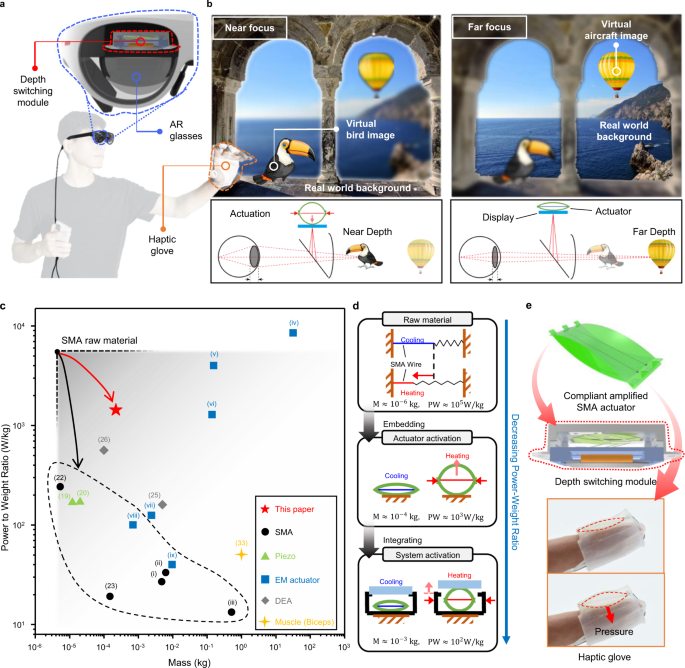The image features a detailed diagram and several photographs against a solid white background, providing an in-depth look at augmented reality (AR) technology. In the top portion, there's a labeled "Depth Switching Module" and an illustration resembling a helmet, which is identified as AR glasses. A man wearing these glasses and haptic gloves is depicted, highlighting the interaction capabilities. To the right are two panels demonstrating the AR experience: the left side (labeled "near focus") shows a vibrant virtual bird perched in an arched window, set against a real-world ocean backdrop featuring a pelican and a hot air balloon. The right panel (labeled "far focus") presents a clearer real-world background with a virtual aircraft image. Descriptive text details technical aspects like a compliant amplified SMA actuator and the depth-switching module, explaining how these components integrate to enhance visual depth perception. Various arrows and labels in black and red further clarify the diagrams. At the bottom, additional charts and graphs provide more context on the technological underpinnings of the AR system.